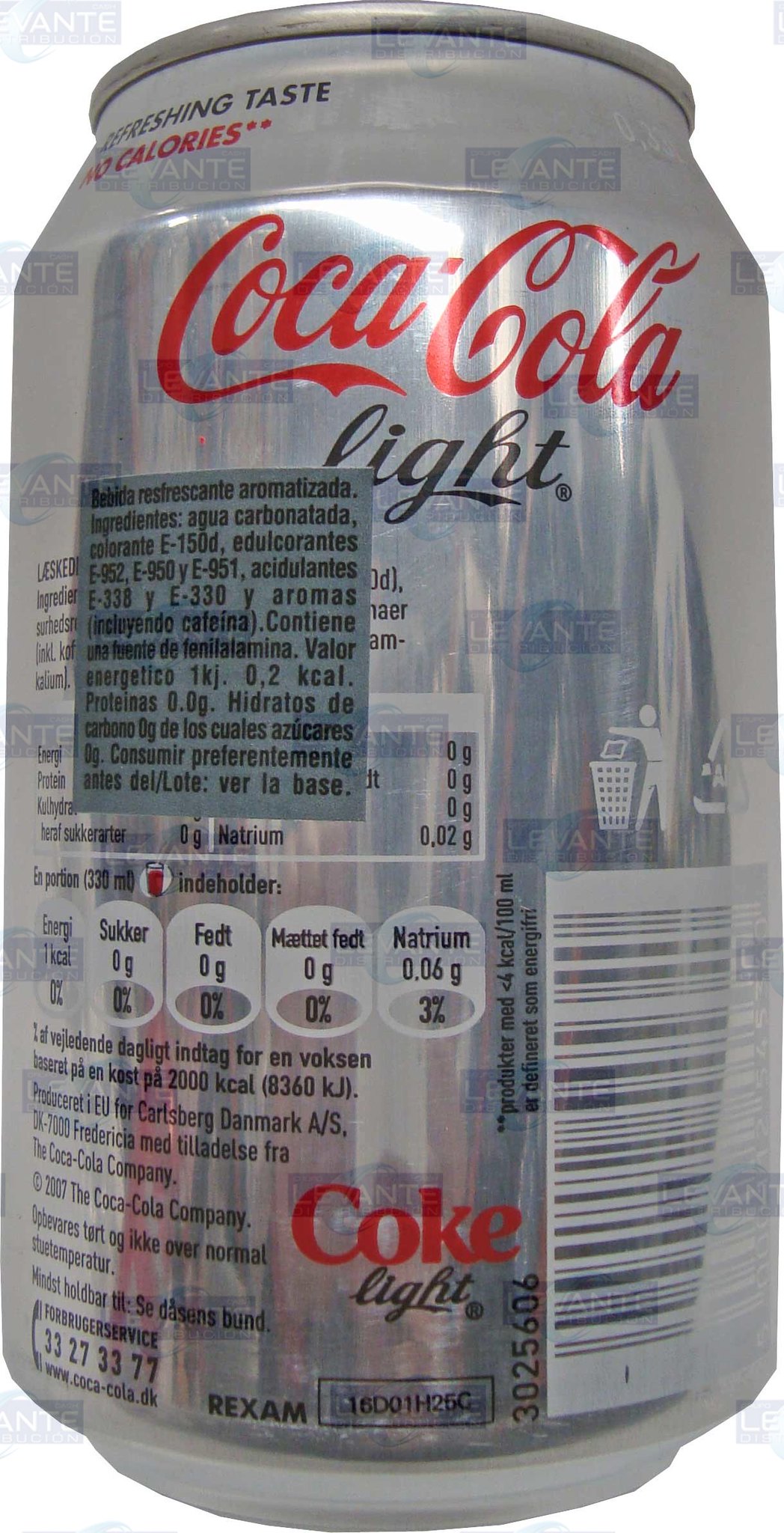This image features a can of Coca-Cola Light, characterized by its sleek silver aluminum exterior. Prominently displayed across the center is the iconic "Coca-Cola" logo in vibrant red, beneath which the word "light" appears in elegant black lettering. The left side of the can is adorned with nutritional information that extends vertically, written in a non-English language, possibly for an international market. On the right side, a white barcode is noticeable, providing precise product identification. Additionally, at the top left of the can, the phrases "refreshing taste" and "no calories" are clearly printed, emphasizing the beverage's appealing qualities.